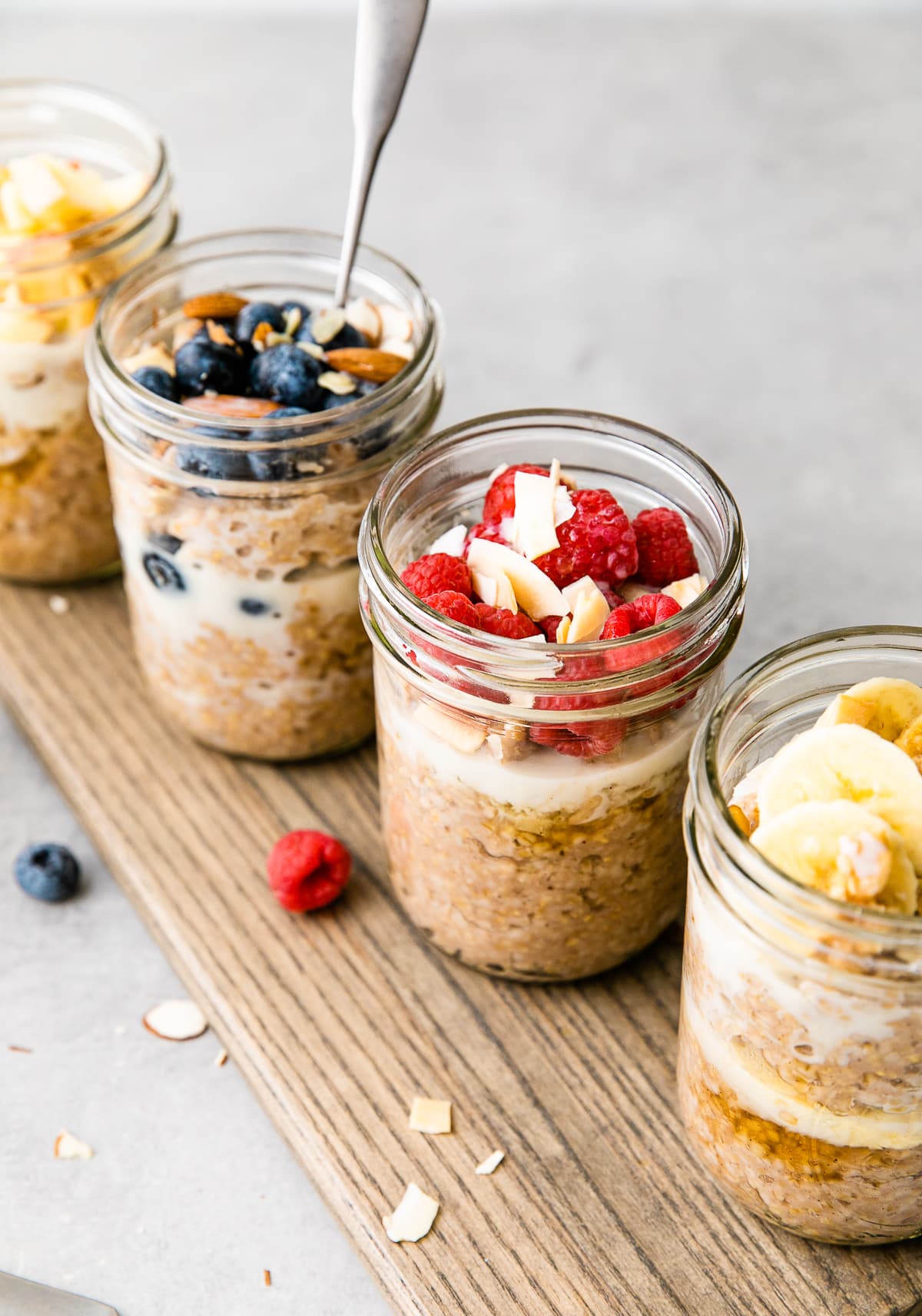This vertically rectangular, full-color photograph features a meticulously staged arrangement of four clear mason jars containing layered parfaits, prominently displayed atop a narrow wooden board with visible horizontal grains. The background is a solid grey countertop, enhancing the rustic appeal of the set-up. The jars are filled with a tantalizing mix of granola at the bottom, a layer of creamy yogurt, and topped with a variety of fresh fruits. 

From right to left, the jar on the far right contains sliced bananas, the one towards the center-right is adorned with raspberries, while the middle jar features blueberries along with a spoon inside. The jar on the upper left side is slightly out of focus and topped with a yellow fruit, potentially bananas or peaches. Scattered around the jars on the wooden board and countertop, are sliced almonds, a single raspberry, a single blueberry, and small bits of granola, adding to the visual appeal and textural contrast of the composition. No text or words are included in the image, keeping the attention solely on the vibrant colors and appetizing display of the parfaits.